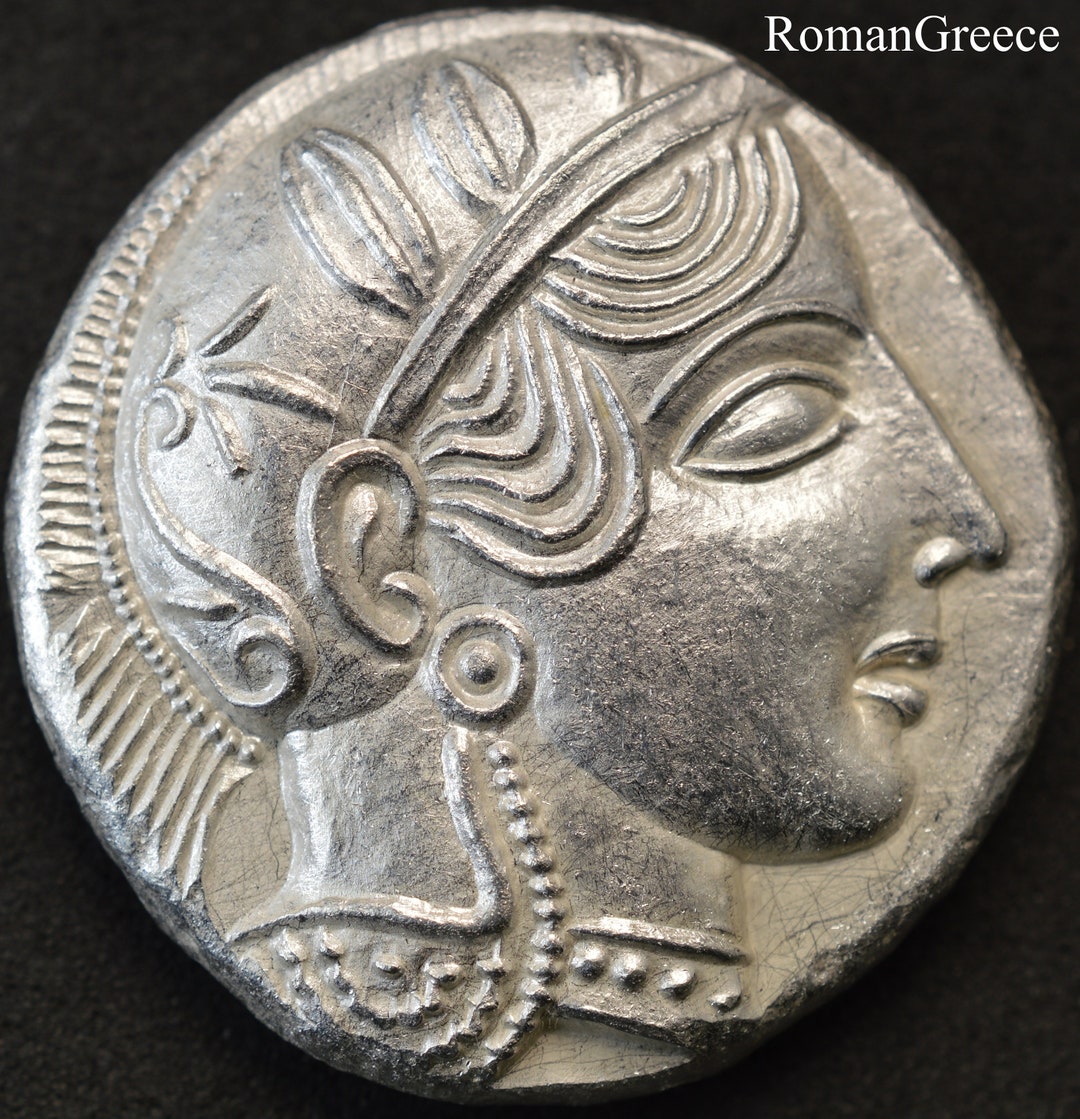This image prominently features an ancient coin, likely of silver composition, set against a square backdrop. The coin itself is round, or nearly so, and showcases intricate craftsmanship. In the upper right corner of the square, the label "Roman Greece" is clearly displayed, suggesting both the cultural and historical context of the artifact.

The focal point of the coin’s design is the right-facing profile of a person, presumably of significant historical or mythological importance. Adorning the person’s head is an elaborate headband interwoven with detailed leaves, which together suggest a laurel wreath—a symbol of victory and honor. The flowing hair beneath the headgear adds a sense of movement and realism to the portrayal. 

Additionally, resting atop the person’s head, there appears to be a depiction reminiscent of a warrior's shield, further emphasizing the martial or heroic nature of the figure. Around the neck, the person wears an ornate collar embellished with studs and beads, intricately wrapping around and enhancing the overall regal and authoritative aura of the representation.